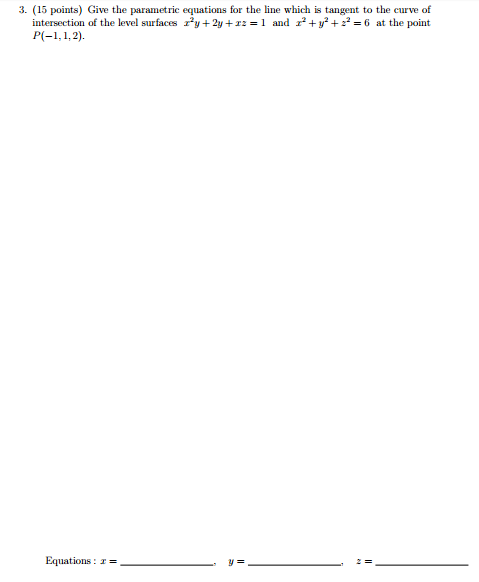The image features predominantly white space, designed to facilitate ample workspace for solving a complex mathematical problem. In the top corner, there is the number "3" followed by "(15 points)" in parentheses. Below that, the problem statement reads:

"Give the parametric equations for the line which is tangent to the curve of intersection of the level surface \(x^2y + 2y + x^2 = 1\) and \(x^2 + y^2 + z^2 = 6\) at the point \(P(-1, 1, 2)\)."

The majority of the page remains blank, intended to provide room for detailed derivations and calculations necessary to solve the problem. At the bottom of the page, there are lines labeled "x =", "y =", and "z =", each providing a line for writing out the final parametric equations. This setup indicates that the assignment is designed to evaluate the solver's ability to handle a detailed and challenging mathematical problem, emphasizing the process and clarity of problem-solving steps.